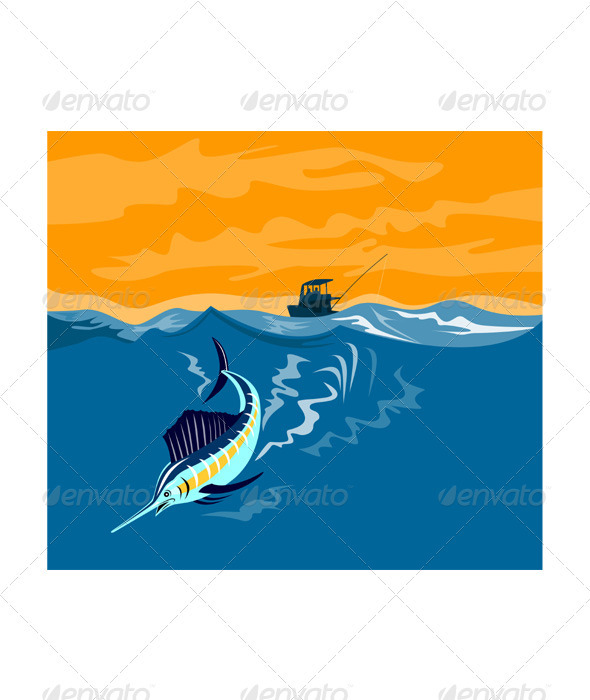This image is an animated seascape featuring a striking scene of a vivid orange-hued sky seamlessly merging with the ocean. The water exhibits various shades of blue, interspersed with dynamic waves and white caps. Centered in the foreground is a swordfish, distinguished by its long, needle-like nose and a light blue body accentuated by a central yellow-orange stripe. The fish's body is further marked with white vertical stripes covering approximately 80% of its length, and it boasts a prominent dark navy-blue dorsal fin.

In the background, a dark blue fishing boat can be seen, equipped with a long fishing rod extending outward, adding to the scene's dynamic narrative. The swordfish appears to be swimming away from the boat, moving toward the left bottom corner of the image. The sky above features whimsical, lighter orange swirls and creatively drawn clouds, enriching the overall animated aesthetic.

A watermark consisting of intersecting grey lines forming diamond shapes overlays the image, with the word "Envato" prominently displayed in text at points where the diamond lines meet, suggesting it is the rightful owner of this visually captivating seascape.